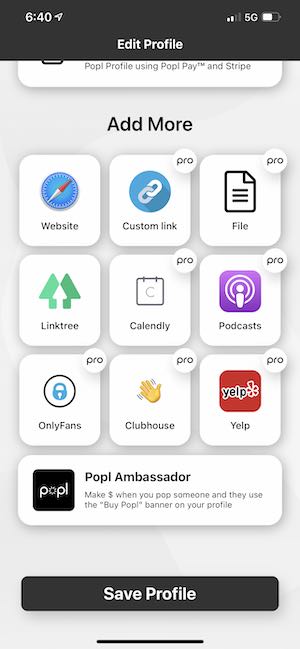This image is a detailed screenshot of a smartphone interface. At the top, a wide black header bar features essential status indicators. In the upper left-hand corner, the time is displayed in white text as "6:40." On the upper right-hand corner, the signal strength is shown with "2 out of 4 bars," accompanied by "5G" connectivity status and a battery icon indicating approximately half charge. The center of this header bar prominently reads "Edit Profile."

The main screen has a very light gray background. Centrally positioned at the top, the text "Add More" serves as a heading. Below this, there are 9 small boxes arranged in a grid, each labeled with different functionalities or platforms: Website, Custom Link, File, Linktree, Calendly, Podcasts, Onlyfans, Clubhouse, and Yelp. Some of these boxes feature a small "Pro" circle in the upper right-hand corner, indicating premium features.

A pop-up or text bar beneath these boxes reads "POPL Ambassador," with a logo to the left. This is followed by a description: "Make Money when you pop someone and they use the Buy Pop banner on your profile."

At the bottom of the image, a prominent wide Save Profile button stands out, with white font on a black background. Further down, centered at the very bottom, is a thin horizontal black line, likely part of the smartphone's user interface for navigation or additional options.